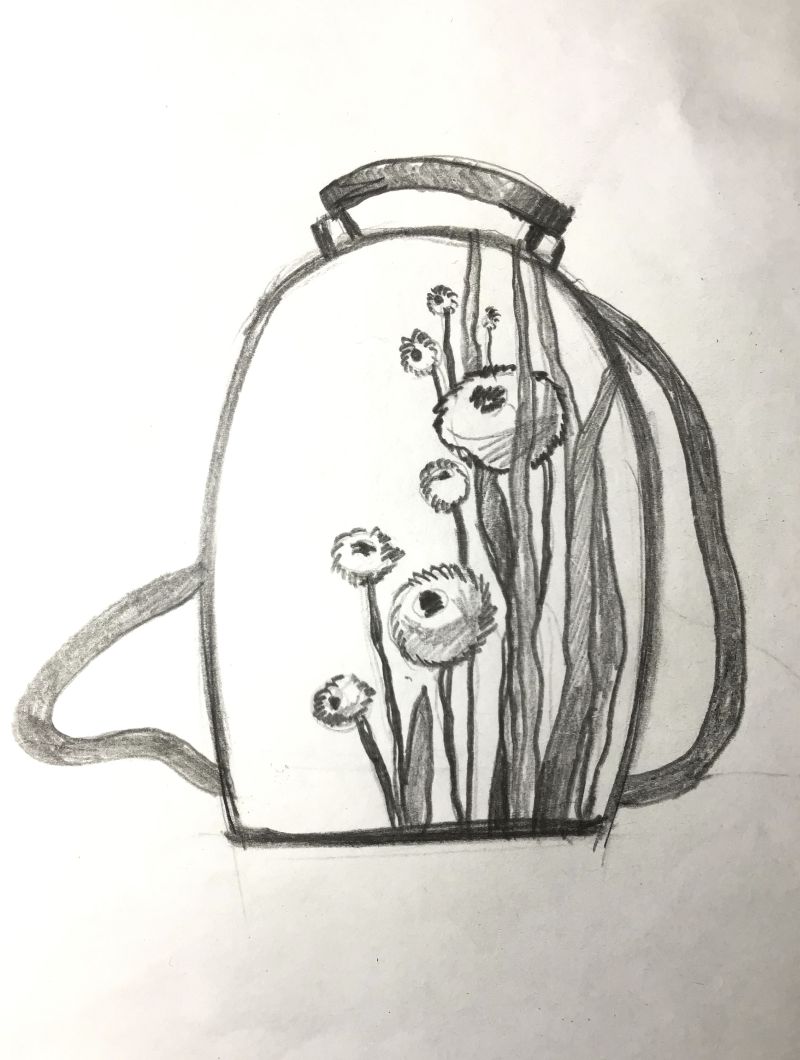This intricate pencil drawing, set against a pristine white background, features an overturned coffee cup as its central element. The cup is depicted with a horizontal dark line forming its base, from which vertical lines ascend, converging at the rounded top. Inside the confines of the cup, on the right side, are delicately drawn flowers with jagged-edged petals and dark circular centers. Surrounding the blooms are leaves and stalks, meticulously shaded to bring out their texture.

Adjacent to the top right edge of the cup, a thick, shaded line gracefully loops down in a backward 'C' shape, seamlessly connecting back at the cup's base. On the bottom left side, another shaded line extends diagonally upwards to the left, then transitions into a horizontal line before curving straight up and over to the right, where it reconnects with the cup structure.

Crowning the composition is a prominently shaded arching banner, its dark tones accentuated by two supporting lines extending downwards to join the main shape on both the left and right sides. The overall effect is a harmonious blend of geometric precision and natural elegance, skillfully rendered in pencil.